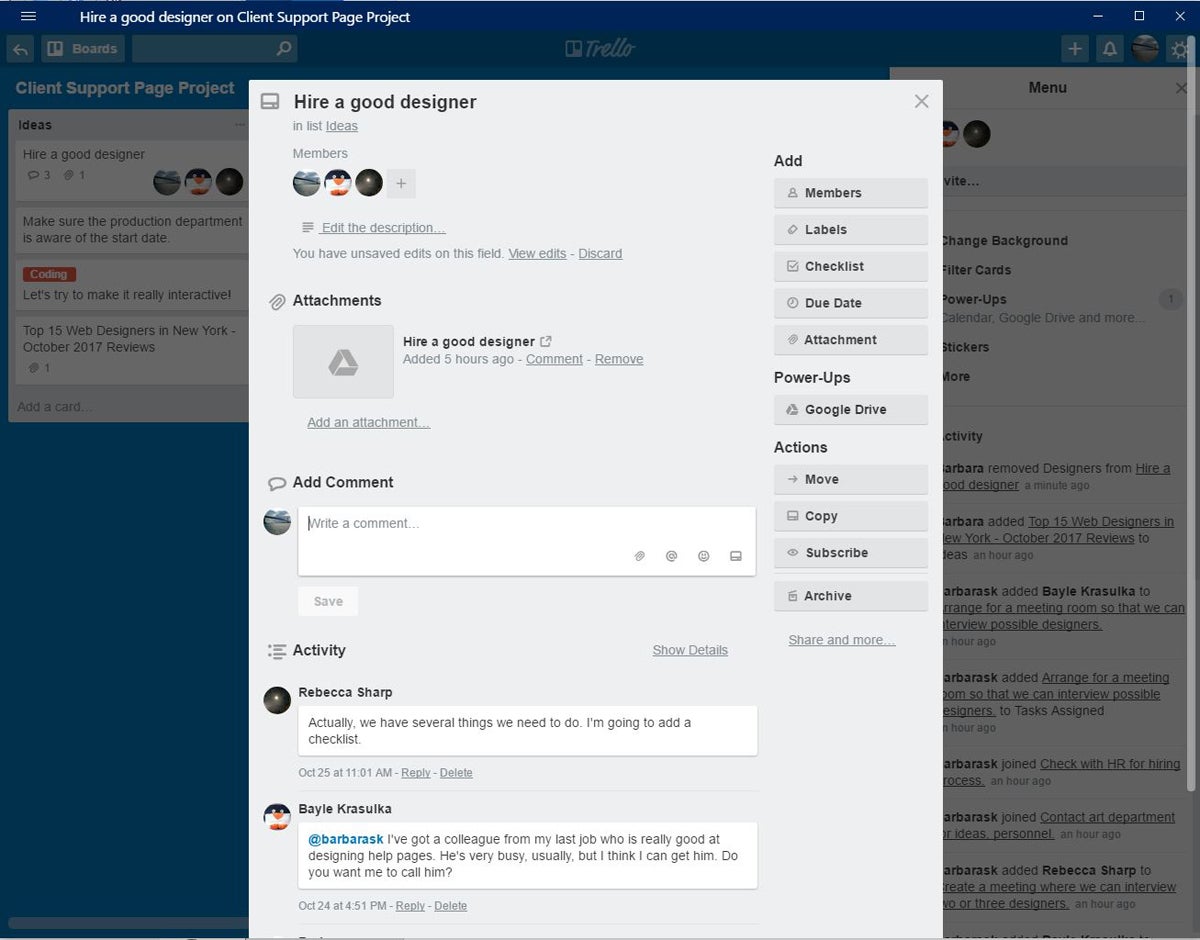The image depicts a website's client support page featuring a project titled "Hire a Good Designer." The top-left corner of the page houses the project title, adjacent to a menu icon consisting of three horizontal lines. The background of the page is a blue gradient with a gray overlay, adding a muted effect.

A prominent gray pop-up window is visible, reiterating the project title "Hire a Good Designer" in the upper left corner. The pop-up includes a section titled "Ideas," with the word "Ideas" underlined. Below this, there is a "Members" section displaying three circular profile pictures and a plus sign for adding more members.

Further down, the pop-up has an "Edit the Description" option followed by a notification stating, "You have unsaved edits on this field," with "View Edits" and "Discard" both underlined. The "Attachments" section lists recent activities, such as the addition of an attachment titled "Hire a Good Designer," added five hours ago, with options to comment or remove also underlined.

At the bottom of the pop-up, there are fields for adding attachments and comments. A data field labeled "Write a comment" is available for user input, accompanied by a gray "Save" button with gray font. The "Activity" section follows, featuring an entry by Rebecca Sharp, who mentions adding several tasks to a checklist. This entry is timestamped October 25 at 11:01 a.m.